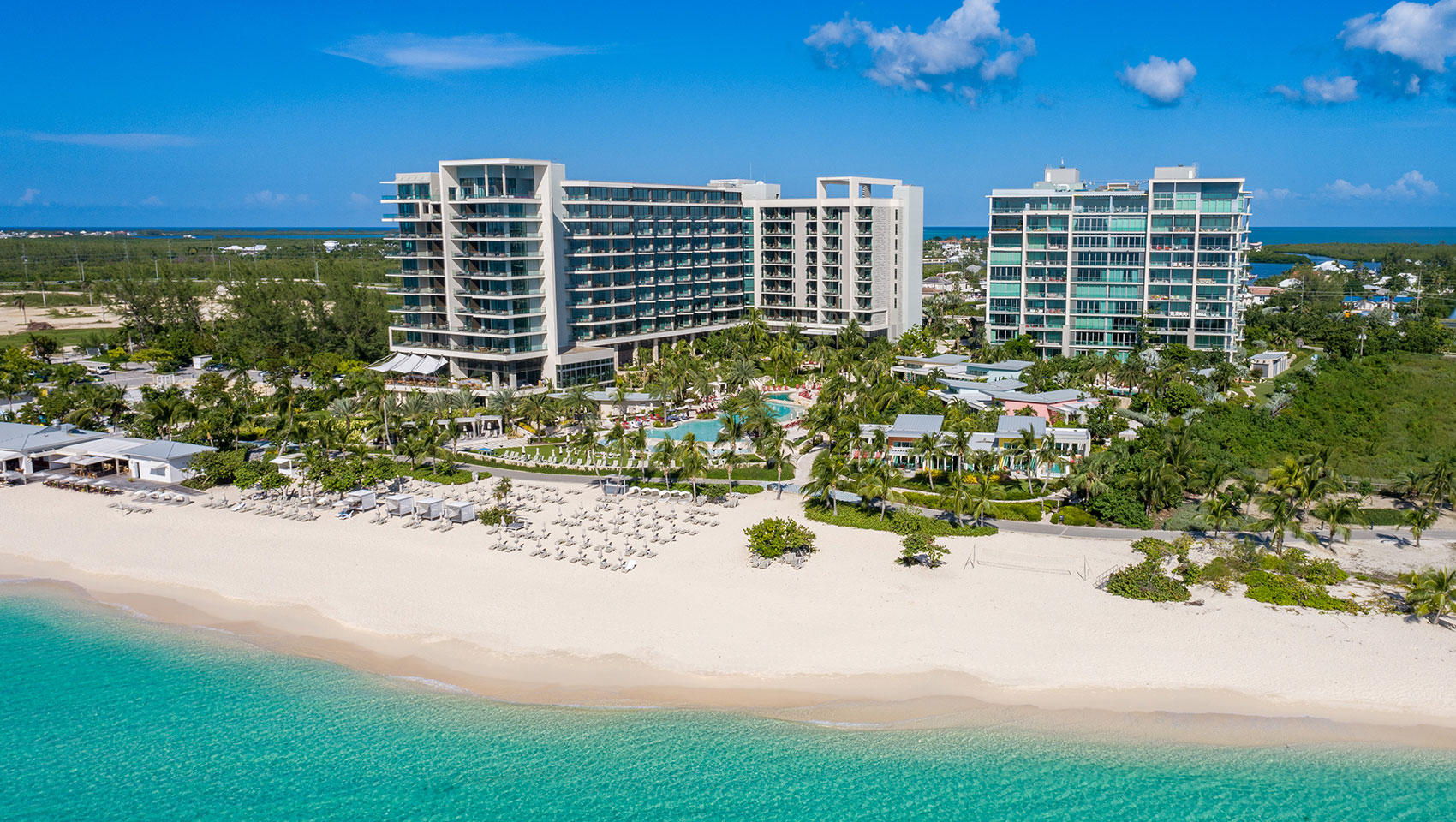A stunning aerial shot captures a picturesque beach scene. The foreground reveals the gentle aqua waves lapping onto the pristine white sand, illustrating the tide's reach. The beach is dotted with the lush greenery of scattered trees, creating a serene contrast to the sandy shoreline. Dominating the scene are two resort buildings; the larger one is a striking gray concrete structure adorned with numerous windows and terraces. Nearby, the smaller building mirrors its architectural style. In front of the resort, several rows of neatly arranged beach chairs invite relaxation. Nestled within the resort complex is a charming kidney-shaped pool, surrounded by smaller buildings, enhancing the idyllic vacation atmosphere.